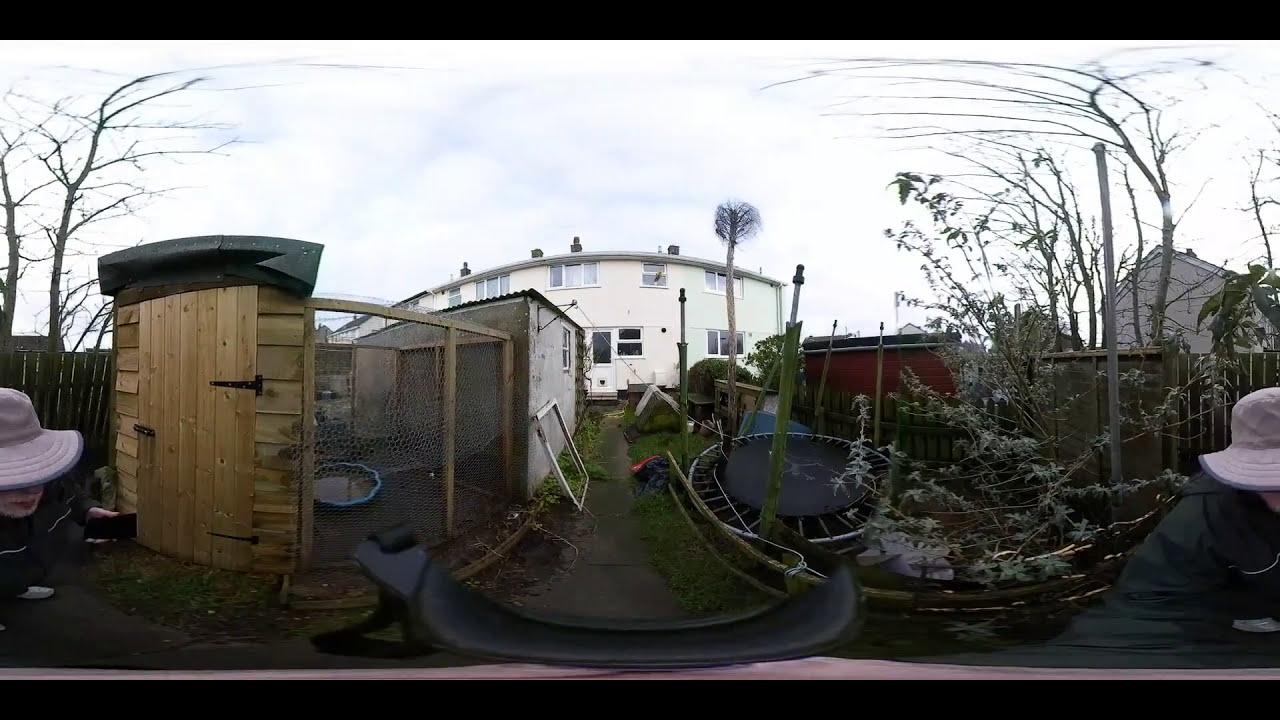The image captures an outdoor scene of a seemingly cluttered yard or garden that resembles a farm-like setting. Dominating the background of the photo is a long two-story white house with a flat roof, surrounded by various elements. In the foreground, a woman, appearing to be of Caucasian descent, is positioned on the lower left side, wearing a wide-brimmed pink hat with a gray outline and a dark greenish-gray jacket with white pinstriping. She is holding a cell phone in her left hand. On the right side, another figure, possibly a man or the same woman due to manipulation of the image, is seen in a green jacket and a white hat with a blue brim, working in what seems like a garden with reed-like plants.

A sidewalk pathway runs from the bottom of the image to the midline, directing attention to the house in the center. To the left of the pathway, a wooden fence with two barren trees stands behind the woman. On the right side, there is an outdoor trampoline next to some mostly barren trees or bushes. Adjacent to the trampoline is a large wooden shed or barn-like structure, its door leading to a chain-link enclosure. Inside this enclosure, a blue child's kiddie pool filled with murky water can be seen, possibly part of a chicken coop. The overall atmosphere suggests a rural or semi-rural home setting, with various elements indicating the presence of animals and gardening activities. The image appears to utilize a 360-camera effect, causing the edges to curve and creating a panoramic view of the entire yard.